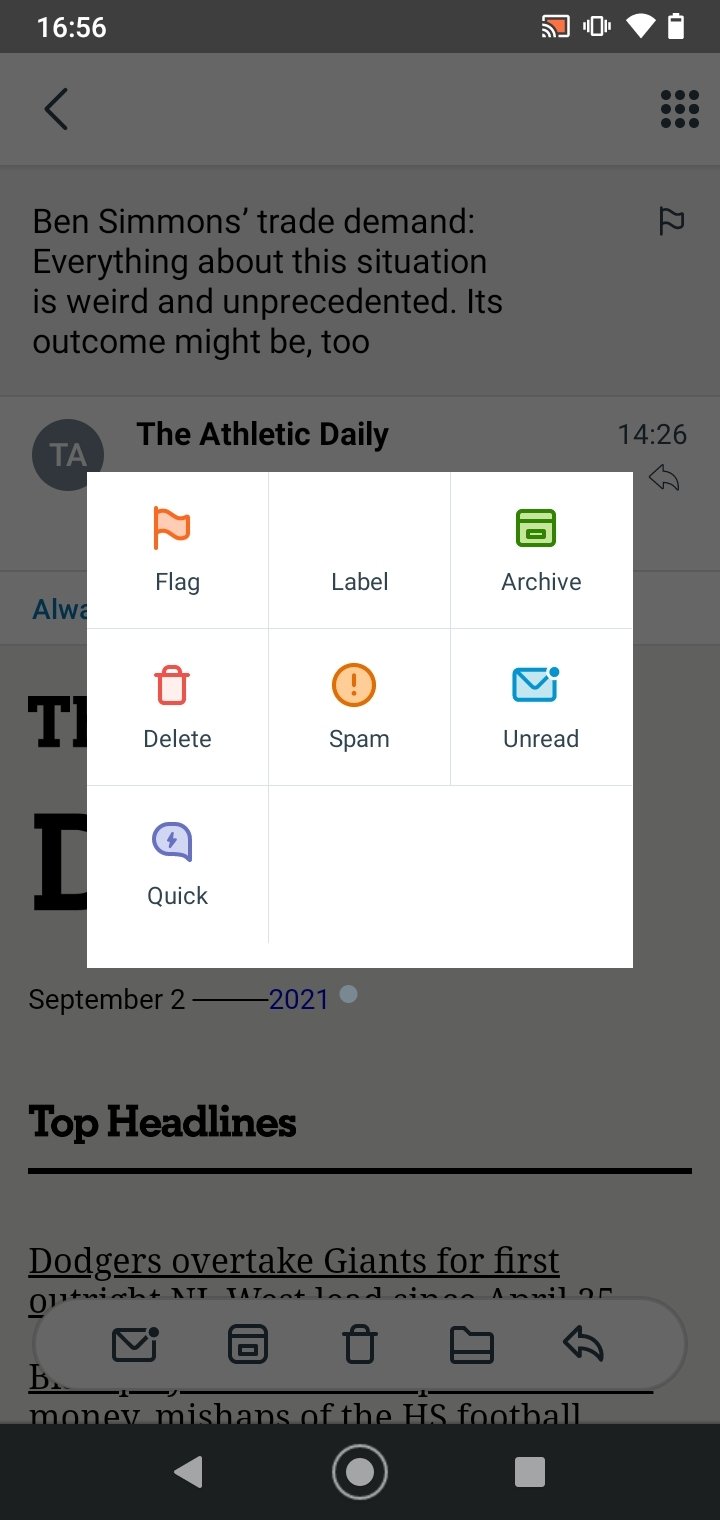In the image, set against a muted gray background, we see a cell phone screenshot showcasing a news article. At the upper left corner, displayed on a black header in white text, is the time '16:56'. On the upper right, icons indicate that the Wi-Fi is active and provide a battery status. Beneath this header, a gray banner contains a navigation menu featuring a 'three dots' icon in three rows, along with a left-pointing arrow. Adjacent to these icons, the headline "Ben Simmons Trade Demand" is boldly presented in black text.

The headline is followed by a subtext stating, "Everything about this situation is weird and unprecedented. Its outcomes might be too," portraying the unusual nature of the trade demand.

Further down, a gray circle with the initials 'TA' in white text marks the logo of 'The Athletic.' To the right of this circle, 'The Athletic Daily' is prominently displayed in bold black text, accompanied by a timestamp reading '14:26'. 

At the bottom of the screenshot, in bold black text, the phrase "Top Headlines" appears, underlined by a thin horizontal black line, indicating the section of the news article.